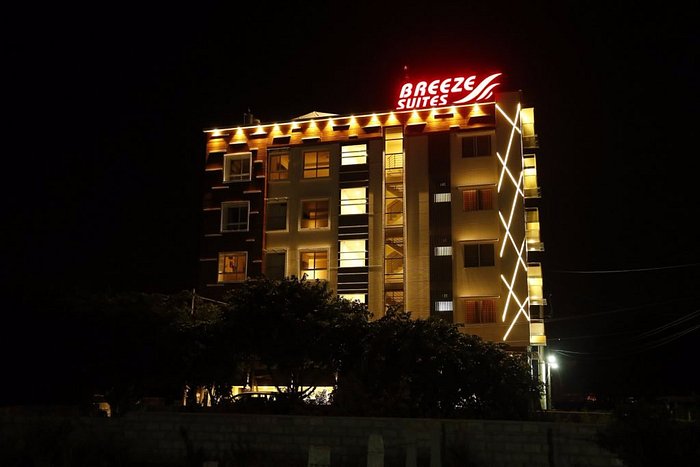This photograph, taken at night, captures the striking image of a hotel called Breeze Suites. The sky is pitch black, with no stars or a moon visible, enveloping the surrounding area in total darkness. In the middle ground, faint outlines of trees are visible in front of the building. The hotel itself appears to be five or six stories tall and is brightly illuminated with yellow and orange lights, highlighting its structure. At the very top of the building, a prominent neon red sign displays the name “Breeze Suites,” accompanied by a wave-shaped logo. The façade features crisscross light patterns, adding to the building’s visual appeal. A set of stairs is visible in the central breezeway, and although the hotel is well-lit, the details of the trees and surroundings remain indistinct due to the enveloping darkness.